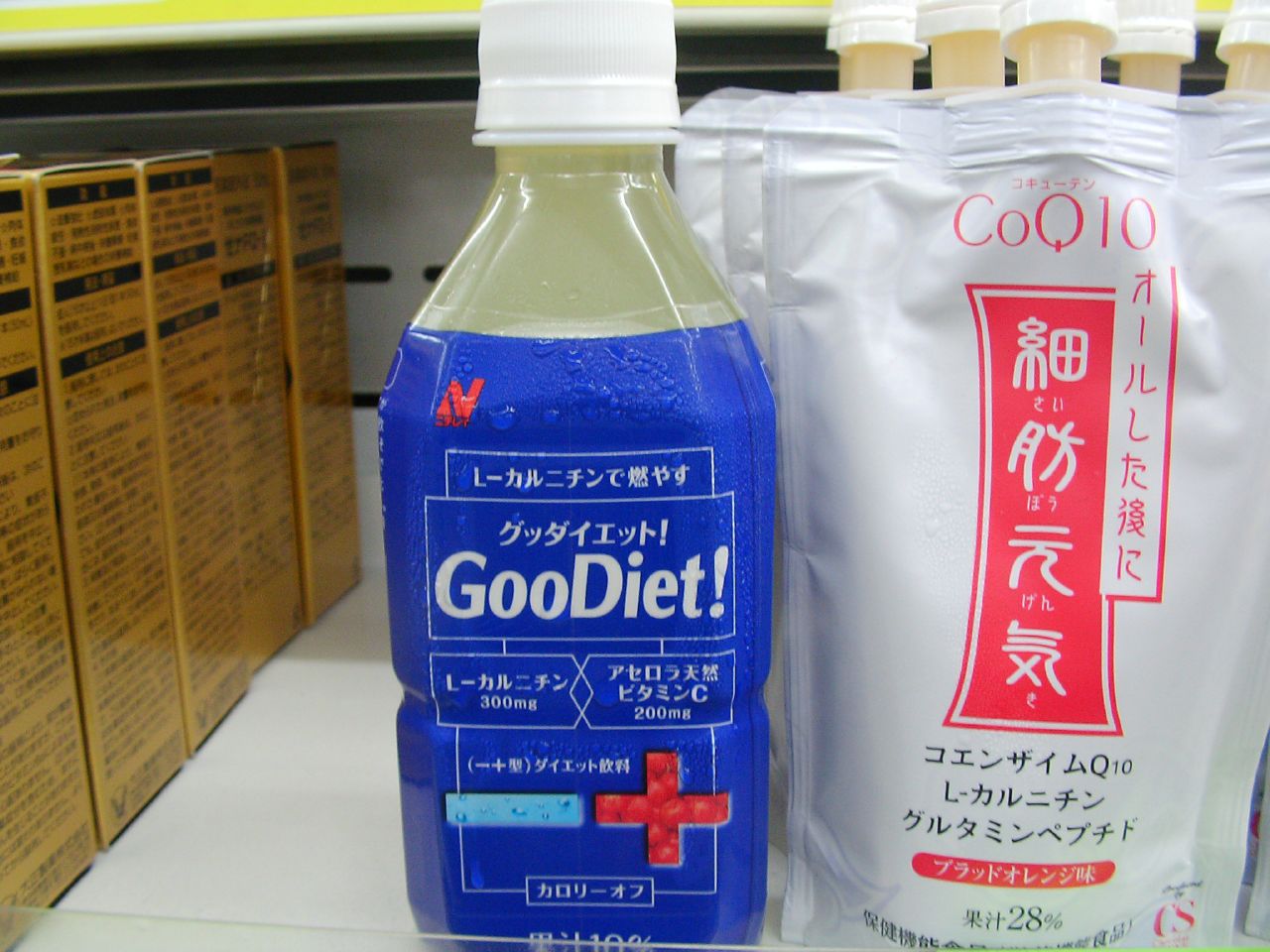This photograph captures an extreme close-up of a store shelf stocked with various products. On the left side of the image, a portion of yellow boxes is visible. These boxes, aligned in a row, feature tiny black Asian text, although their full labels are obscured by the edge of the photograph. The shelf itself appears to be a standard plastic or metal fixture commonly found in grocery stores. 

On the right side of the frame, a variety of white packages are prominently displayed. These packages, which seem to be pouches, wrap around bottles with white caps. Inside the bottles, the liquid appears orange in color. The white pouches are marked with both red and black Asian text, alongside a red banner, though the specific contents remain unclear. Next to these pouches stands a clear plastic bottle with a white cap and a blue label. The label, primarily in Asian text, includes the English words "Goo Diet" and small numerical details such as "300mg," "200mg," and percentages like "28%". The liquid inside this bottle appears cloudy and somewhat similar to the color of diluted orange juice or urine. This bottle and packaging ensemble creates a visually compelling segment of the store shelf, rich with diverse products marked by intricate labeling.